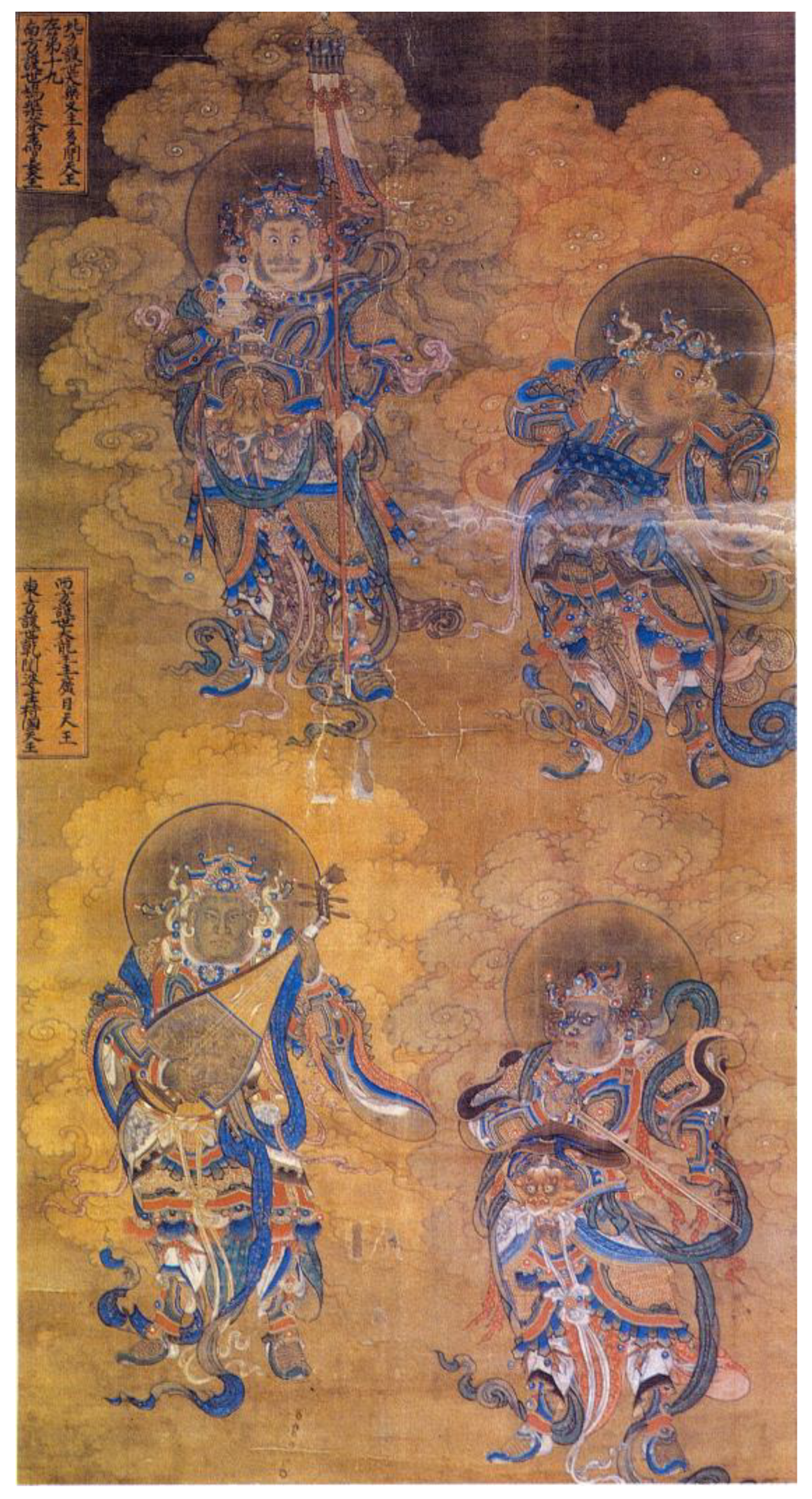This tall, faded, and weathered painting, resembling an ancient Asian artwork on parchment, showcases four opulently dressed figures arranged side by side, two at the top and two at the bottom. Each figure wears flowy, ornate clothing adorned with intricate blue and orange patterns, and swirling ribbons or scarves embellish their attire. The figures have indistinct body shapes and are depicted either looking forward or to the sides, with moons behind their heads. Surrounding them are illustrations of serpentine patterns and small royal blue balls. The background features smoky orange and brown tinted clouds, subtly varying in shades of yellow, orange, and blue. On the left side of the parchment, there is Chinese or Japanese writing, inscribed in black within rectangular boxes.